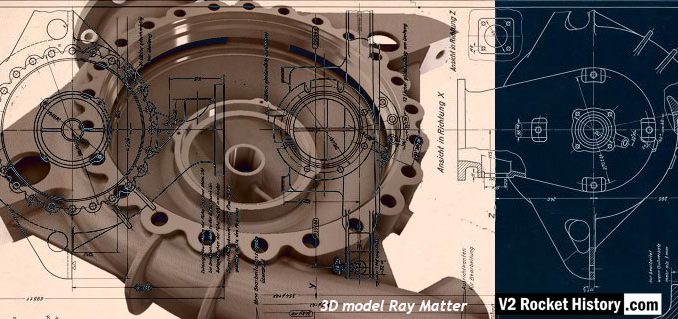The image is a detailed, rectangular blueprint or schematic for a 3D model related to a V2 rocket, featuring multiple engineering elements. The background is divided into two parts: the left two-thirds are tan, while the right one-third is dark blue. Over the entire background, various intricate schematics are overlaid, depicting parts such as engines, gears, and fasteners, which seem to serve a decorative purpose rather than providing specific details.

On the left side of the image, there is a prominent gray cylindrical part resembling a turbine casing or bowl-like structure. This part features indentations around its edge and a central hole that appears designed to house a turbine or similar component. Extending from this central piece is a tube or pipe that winds its way from the bottom right towards the top left. The cylinder also has several attachment tabs and horseshoe-shaped elements for securing additional components.

At the bottom of the image, in white text, it reads, "3D Model Ray Matter, v2rockethistory.com." This text indicates the model's name and a website related to V2 rocket history. The right side of the image, within the dark blue section, includes additional diagrammatic lines that run from the upper right to the lower right, creating a nearly circular pattern. Some small text in this area appears to be in German, but it is too small to decipher clearly in the image. Overall, the image effectively merges artistic representation with technical details, highlighting a component of the V2 rocket.